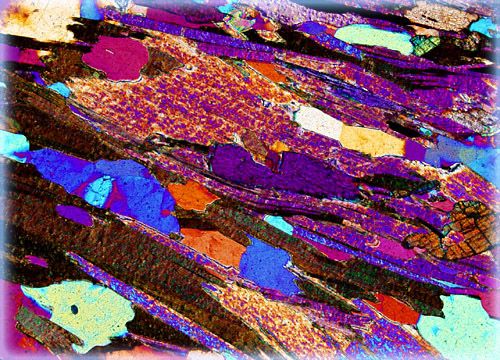This square, abstract painting features a vibrant and dynamic collage of colors, structured to resemble flat, slanting rock formations, akin to shale. Predominantly, the image showcases a cascading arrangement from the top left to the bottom right.

In the **bottom left corner**, you can observe a palette of browns intertwined with light green, purple, and red hues. Moving **upwards towards the middle**, the colors transition to areas rich in blue, orange, and brown tones. **Upper segments** of the painting exhibit a whitish-orange expanse speckled with purple and orange, alongside solid purple streaks. The **top left** corner is distinctly marked by a bright yellow square, adjacent to narrower bands of light and dark purple.

The **bottom right corner** is dominated by white with red and black elements above it, and as we travel to the **top right corner**, a mix of blue, tan, white, purple, and black is prevalent. Central regions of the painting showcase the presence of purple, black, and blue interspersed with yellow, pink blotches, tan, and patches of brown.

Overall, the image is characterized by its splash design with colors ranging from black, brown, purple, light blue, green, orange, and yellow. These colors are energetically smeared or splashed across one another, creating a slightly distorted yet vividly bright and clear setting. No textual or numerical elements are present within the painting.